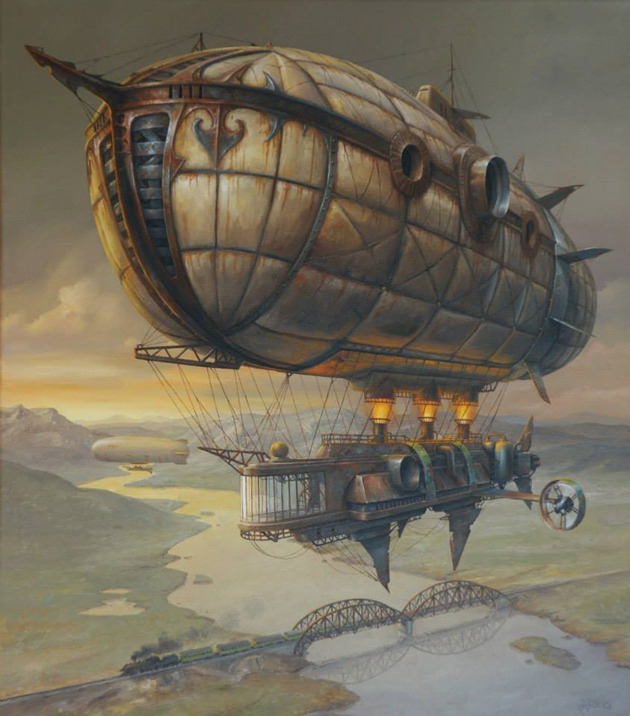The image is a stunning piece of fantasy artwork featuring a fantastical airship as the focal point. This steampunk-inspired airship, with its tan and dark brown hues, resembles both a submarine and an old, rusty pirate ship. The main body of the airship features three visible stacks with bright orange flames contained within glass enclosures, giving it a powerful and almost otherworldly appearance. The passenger section looks metallic and futuristic, yet worn with age. This impressive capsule-like vessel floats high above a serene river, which is spanned by a train trestle. A black train, towing green and gray cars, crosses the bridge located in the lower left-hand corner of the image. Surrounding the scene are vast grasslands and majestic mountains, illuminated by a setting sun that casts a beautiful array of colors—beige, white, rust, brown, red, green, blue, and yellow—across the sky.